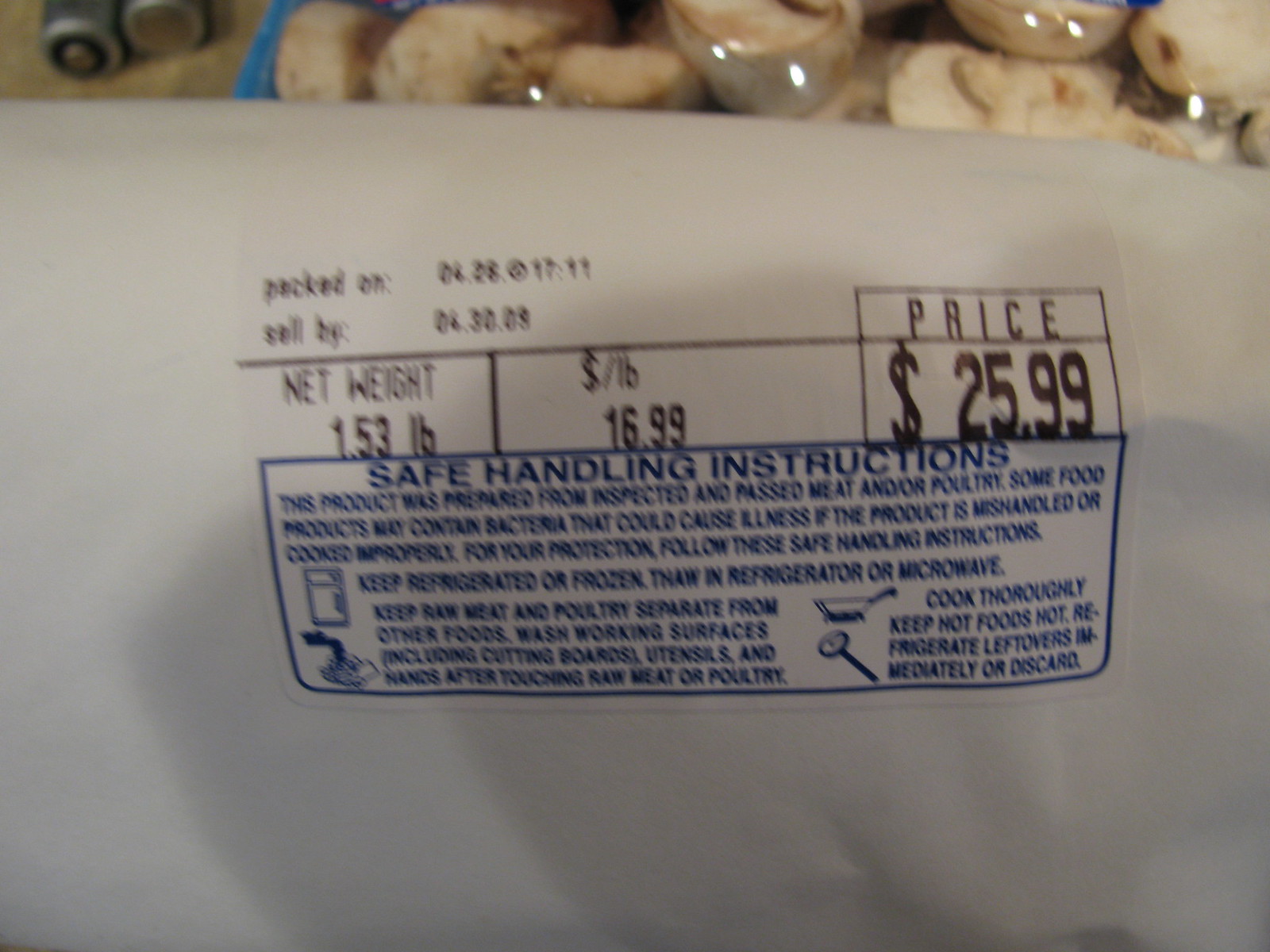The image is a close-up shot of the back of a mushroom bag. The focal point is a white label with various details in small black text, slightly blurry. The label includes the following information: "Packed on: 04.26," followed by a round symbol and "17.11." The "Price per pound" is listed as "$16.99," with a "Net weight" of "1.53 pounds." It also specifies "Sell by: 04.30.08," and the total price is "$25.99." The bag of mushrooms is visible in the background, providing a context to the close-up label.